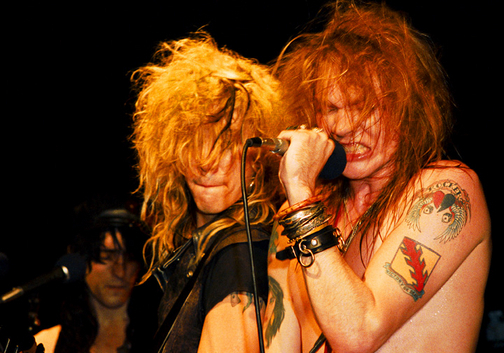This detailed photograph captures an electrifying moment on stage with the rock band Guns N' Roses, likely from the 1980s. Front and center, Axl Rose, with wild, long red hair partially obscuring his face, is fiercely gripping a microphone close to his snarling mouth, his eyes squinched shut in emotional intensity. Axl's muscular arms are showcased by his numerous tattoos, one depicting a woman and another featuring a square symbol with a red feather-like element. He is adorned with several chunky bracelets on his left wrist. Standing closely to Axl, the blonde guitarist, presumably shirtless except for a guitar strap, sports equally disheveled, long hair that covers his face, augmenting his rock 'n' roll aura. He wears a cut-off sleeve black shirt, exuding a raw, rebellious energy. In the background, possibly Izzy Stradlin, with dark hair, a black hat, and a black sport coat, is playing the guitar, while another dark-haired band member is vaguely visible, suggesting the presence of a drummer or a pianist. All band members appear to be of European descent, and the scene is set against a stark black backdrop, emphasizing the dramatic and classic ambiance of this iconic stage performance by Guns N' Roses.